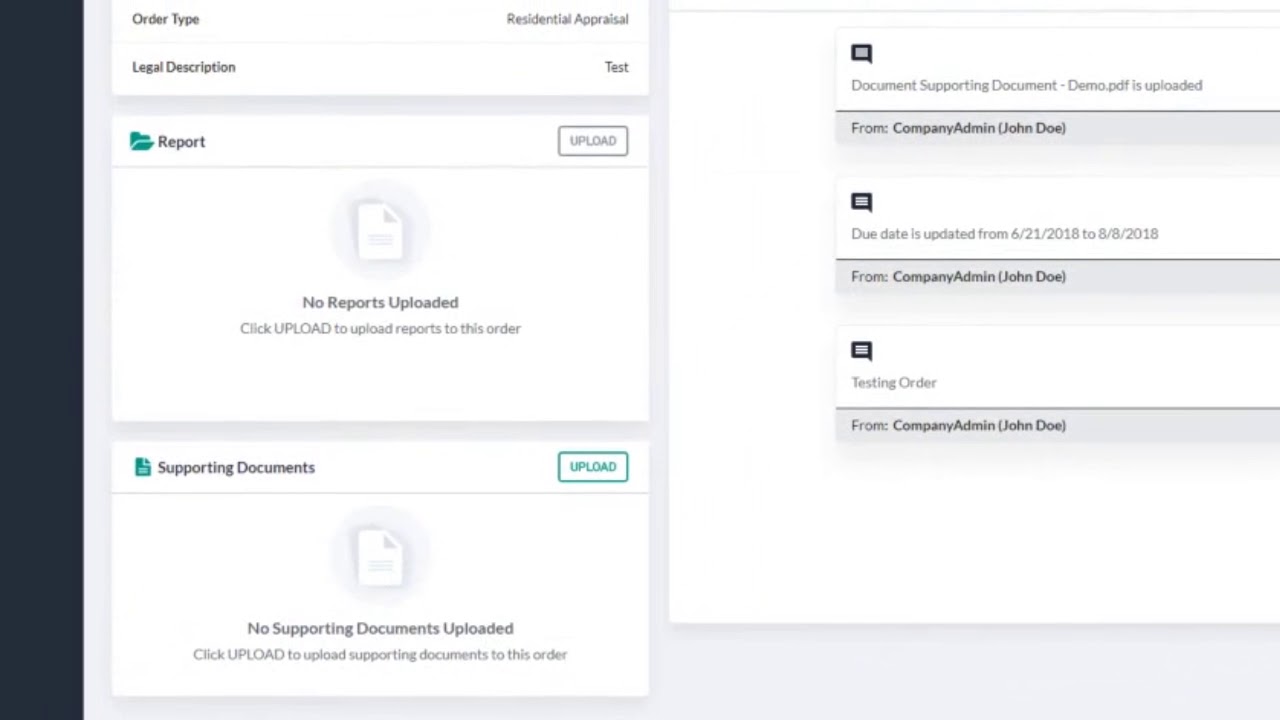In this image, which appears to be captured from a digital device such as a cell phone, tablet, or laptop, we see a detailed workflow chart designed for project management. The chart provides various functionalities and options for handling reports and supporting documents.

At the top of the chart, users have the option to download or add reports directly to the project file, enhancing ease of data handling and accessibility. The interface then transitions to a section titled "Supporting Documents," which offers the functionality to upload additional documents pertinent to the project.

On the far right side of the screen, three distinct options are visible, enabling efficient document management. The first option allows users to send documents directly to a specified individual, in this case, John Doe. The second option details the due dates for document submission, spanning from June 21, 2020, to August 8, 2018. Lastly, there is an option to handle testing orders, which can also be uploaded and managed within the workflow.

Overall, this comprehensive workflow document serves as a central hub for coordinating various aspects of a project. It enables users to upload reports, manage supporting documents, and ensure timely communication with the company administrator, John Doe. The chart facilitates a structured and efficient project management process, keeping all relevant documents organized and accessible.